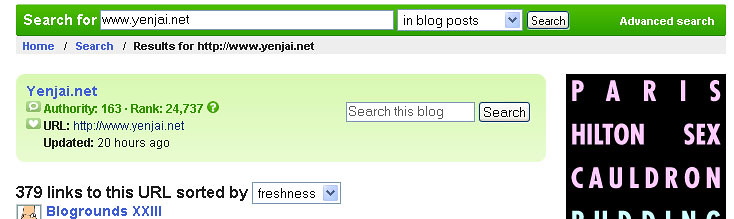The screenshot depicts a website featuring a search bar at the top, into which the user has keyed "www.yenjai.net." Below the search bar, the website displays a light green text box containing the details: "yenjai.net," "Authority 163," "Rank 24,737," and the URL as "http://www.yenjai.net," along with an indication that it was updated 20 hours ago. In bold black font, the text "379 links to this URL sorted by" appears, with a drop-down menu set to "freshness." Below this, in royal green font, the text "Below Grounds XXIII" is visible. On the right side of the image, a prominent black box with bright pink letters reads "Paris Hilton Sex Cauldron." The screenshot gives an overall sense of a disorganized and visually cluttered webpage.